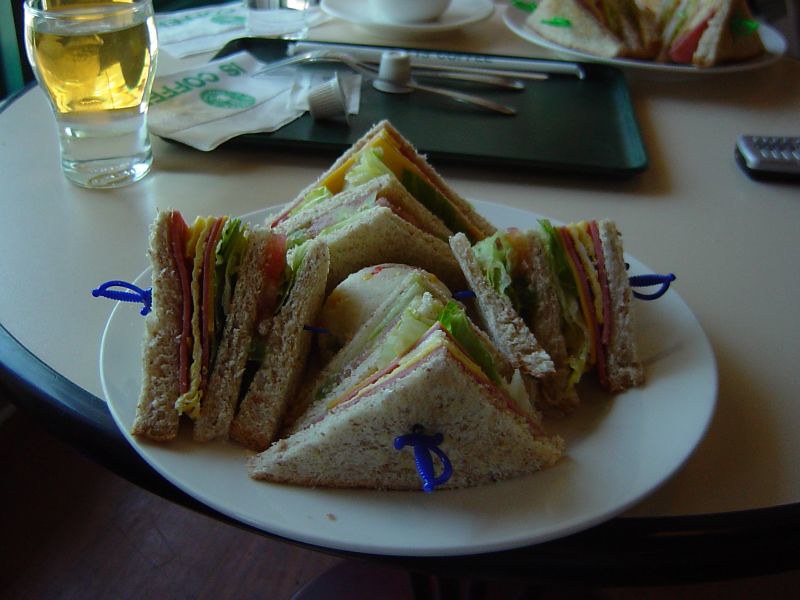In this indoor restaurant photograph, a white circular plate showcasing a meticulously arranged club sandwich dominates the foreground, set on a round table with a beige center and black edge. The sandwich, cut into four triangular sections, features three layers of bread encasing fresh ingredients including lettuce, tomato, cheese, ham, and bacon. Blue plastic sword-shaped toothpicks secure each sandwich piece. A peculiar white circular object, possibly a potato or another item, sits at the center of the sandwich arrangement. 

A clear glass containing a beer, with its rich golden hue, is visible towards the upper left of the image. Behind the plate and slightly out of focus, a dark rectangular serving tray holds various dining utensils including a fork, spoon, knife, and a straw, accompanied by white napkins adorned with green circular prints and the word "coffee." A similar sandwich plate peeks in from the upper right corner, adjacent to a white saucer with a partially visible cup. The photograph, expertly focused on the main plate and beverage, captures the lively yet orderly setting, accentuating the textures and colors of the mouthwatering club sandwich.